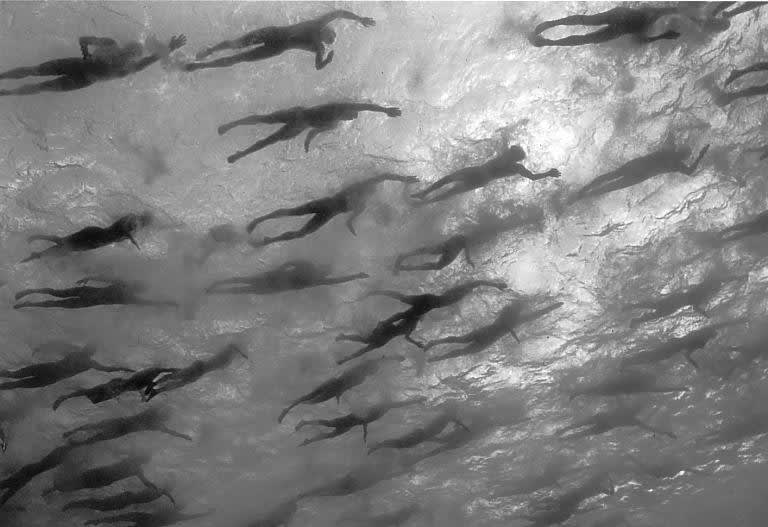This black-and-white photograph captures the dynamic motion of dozens of swimmers, possibly from the 1920s, swimming in unison in a body of water. Taken from beneath the water's surface, the camera looks up towards a scene teeming with activity. The swimmers, appearing as dark shadows against the lighter, shimmering backdrop, seem to be wearing old-fashioned, full-body or long, skin-tight bathing suits, a style typical of the early 20th century. The image, a horizontal rectangle, is dominated by a sense of movement and aquatic turbulence as the swimmers paddle and kick their way across the frame, moving from left to right and slightly upwards. The sunlight breaks through the surface, casting a radiant glow predominantly on the right side of the photograph, highlighting the contrast between the swimmers' dark forms and the surrounding grays and whites. More swimmers are clustered towards the bottom left of the image, adding to the sense of depth and motion in this captivating underwater snapshot.